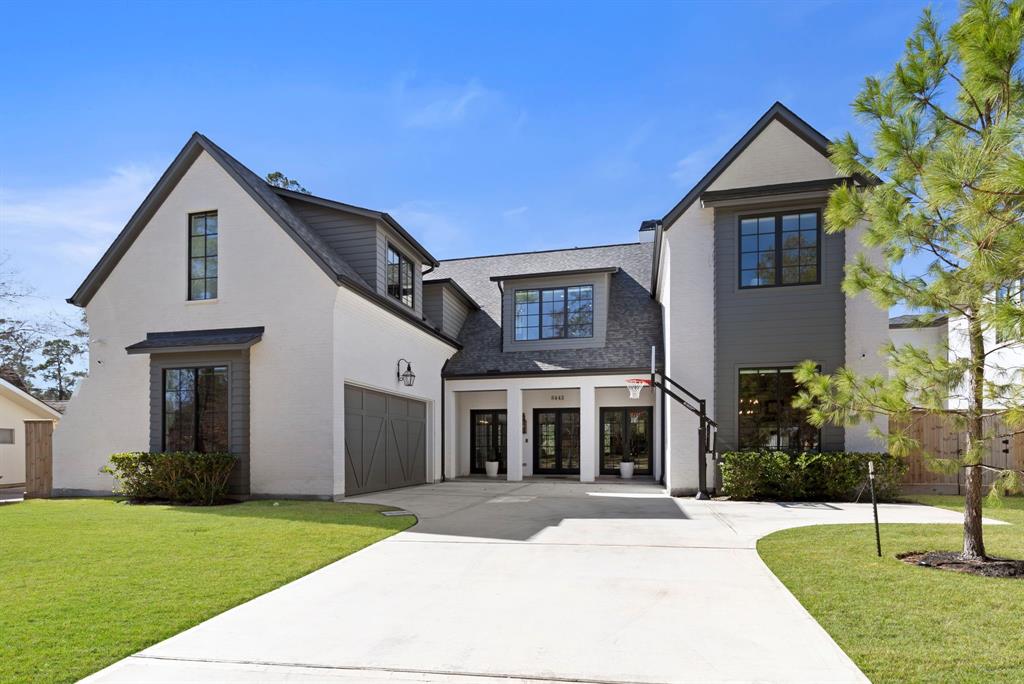This is a detailed photographic image captured outdoors during the day, depicting a fairly large and elegant two-story house. The house features an intricate architectural style, characterized by two sets of gray gabled roofs on the left and right with a connecting gabled roof in the middle, giving the impression of two houses joined by a hallway. The exterior walls are primarily white, accented by gray and some black around the window panes, offering a striking contrast against the bright blue sky dotted with a few wispy clouds.

Central to the image is a pristine concrete walkway leading up to the house. The walkway is flanked by green, well-manicured lawns and bordered by sparse bushes situated in front of tall windows on both sides. One notable tree, which appears evergreen and somewhat sparse, stands prominently to the right of the walkway.

In front of the house, positioned on the right side of the concrete driveway, there is an outdoor basketball hoop complete with a stand and net. The driveway itself is empty, devoid of any vehicles. The front facade of the house features several large windows and three sets of double doors, some leading to sliding doors, with potted plants in white pots accentuating the entry points. Above the central door, slightly blurred and unreadable, is a house number. The overall scene is set against a clear, nearly cloudless sky, making the house and its surroundings appear vividly illuminated by daylight.